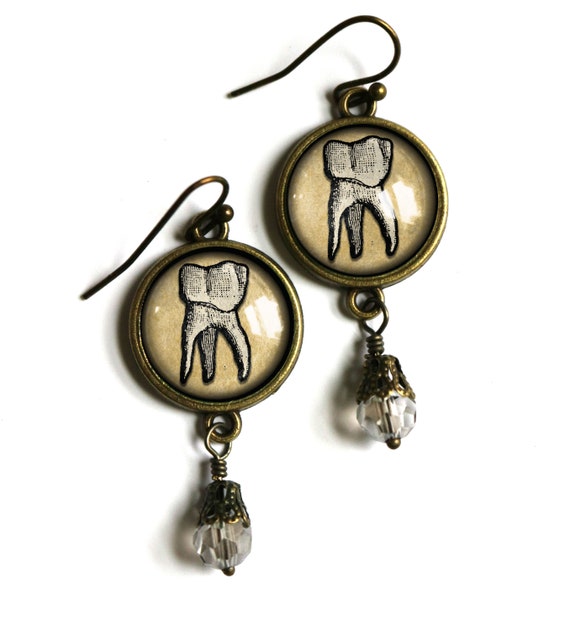This close-up image, taken in portrait orientation, showcases a pair of identical gold earrings laid side by side on a white background. The earring on the left is positioned slightly lower than the one on the right. Each earring features a circular pendant made from a dark gold or brass metal material. The surface of the pendant is smooth and flat, encircled by an outer rim. The central design on the pendant depicts a stylized molar tooth in shades of gray or silver, consisting of a roughly square top with curvilinear lines and three pointed extensions beneath it. Below the main pendant, a smaller circular loop connects to another small circle, from which dangles a clear, crystal-like rock. The earrings have a glossy appearance, with the metal exhibiting a dark brown, bronze-like hue and the hooks designed to be open and insert into the ear.